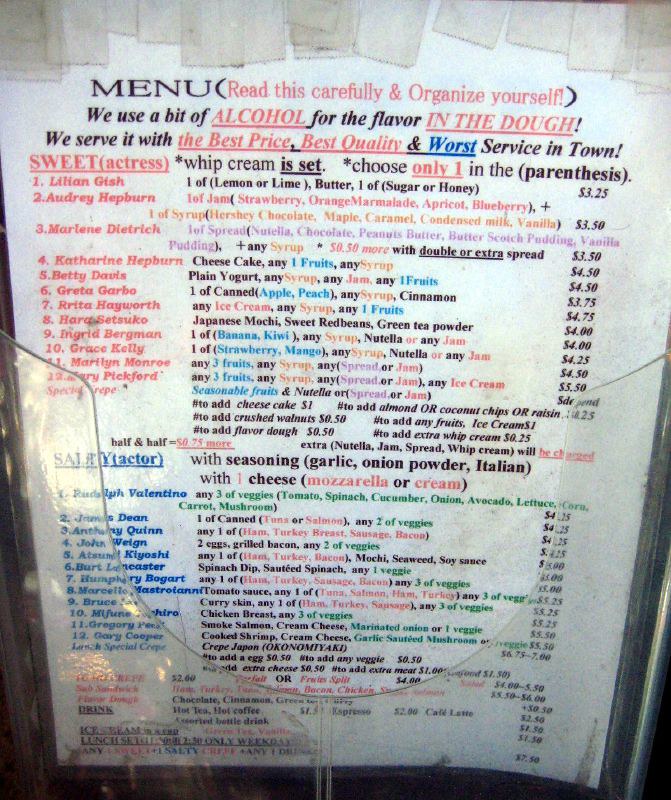This image depicts a highly detailed and unique menu encased in a clear lucite container, which is mounted on a paneled wall of very dark wood. The menu is quite old, evident from the multiple layers of tape mending its worn edges. Despite its age and dinginess, the menu bursts with vibrant colors, with vegetables listed in green, meats in red, and spreads in purple, amongst other hues, making it visually engaging.

At the top, the word "Menu" is prominently displayed in black. Below, there's a playful yet candid advisory urging patrons to "read this carefully and organize yourself," along with a note about using a bit of alcohol for flavor in their dough. The establishment boasts of offering "the best price, best quality, and worst service in town."

Sections for actresses and actors are distinctly highlighted in red and blue, respectively. Famous names such as Audrey Hepburn and Marlene Dietrich grace the actresses' section, while John Wayne and James Dean are listed among the actors. Each name is accompanied by specific prices and descriptions of items, adding a quirky, nostalgic charm.

Though visibly aged and dirty, the vibrant color-coding and the eclectic celebrity-themed dishes lend the menu an undeniable charm, inviting diners to a whimsical and memorable culinary experience.